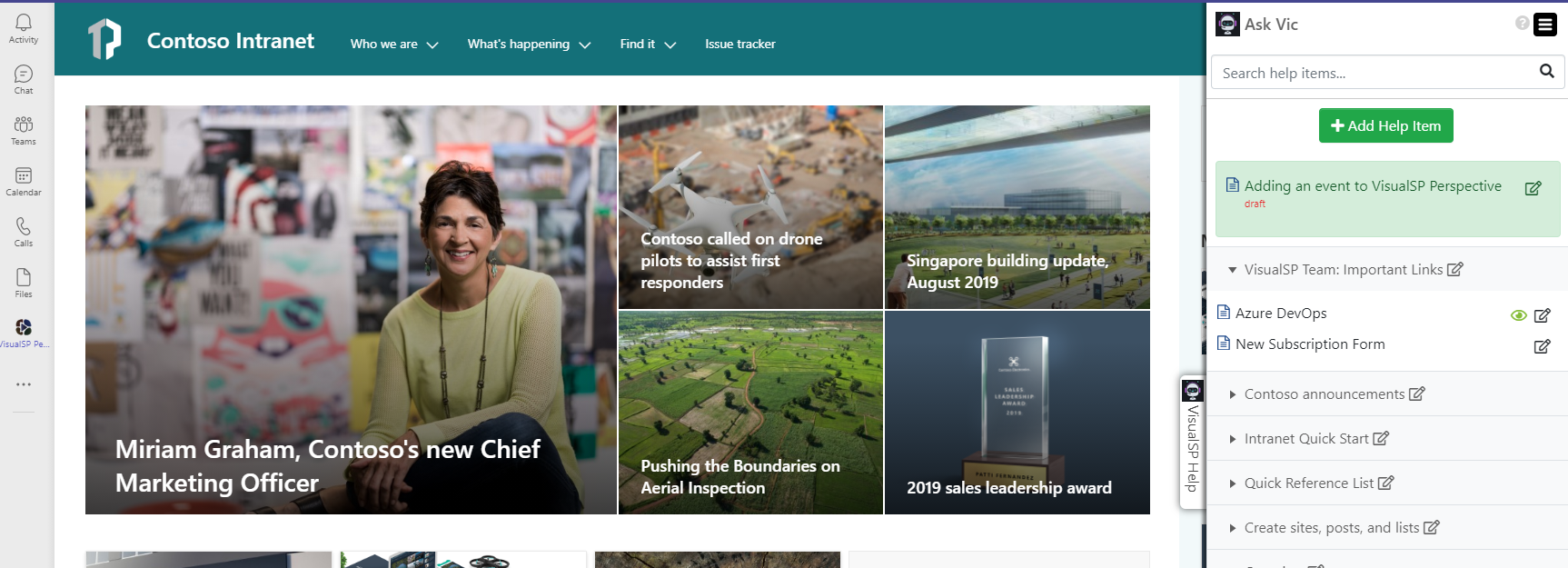This image is a detailed screenshot of the homepage from the Contoso Intranet, which appears to be an internal network for a company or educational institution named Contoso. The header features the Contoso logo, which resembles the outline of a house, although it is not entirely clear. In addition to the logo, the top navigation bar includes links to sections titled "Who We Are," "What's Happening," "Find It," and "Issue Tracker."

The main area of the homepage is filled with a series of headline news articles accompanied by images. The first headline announces "Miriam Graham, Contoso's New Chief Marketing Officer" and includes a photograph of Miriam Graham. The next article, "Contoso Calls on Drone Pilots to Assist First Responders," features an image of a drone in flight. Following this, there is an update titled "Singapore Building Update August 2019," which is illustrated with a conceptual design of a building. Below these articles is the "2019 Sales Leadership Award," highlighted with an image of an award trophy. The final article, titled "Pushing the Boundaries on Aerial Inspection," displays an aerial, almost bird's-eye view of several fields.